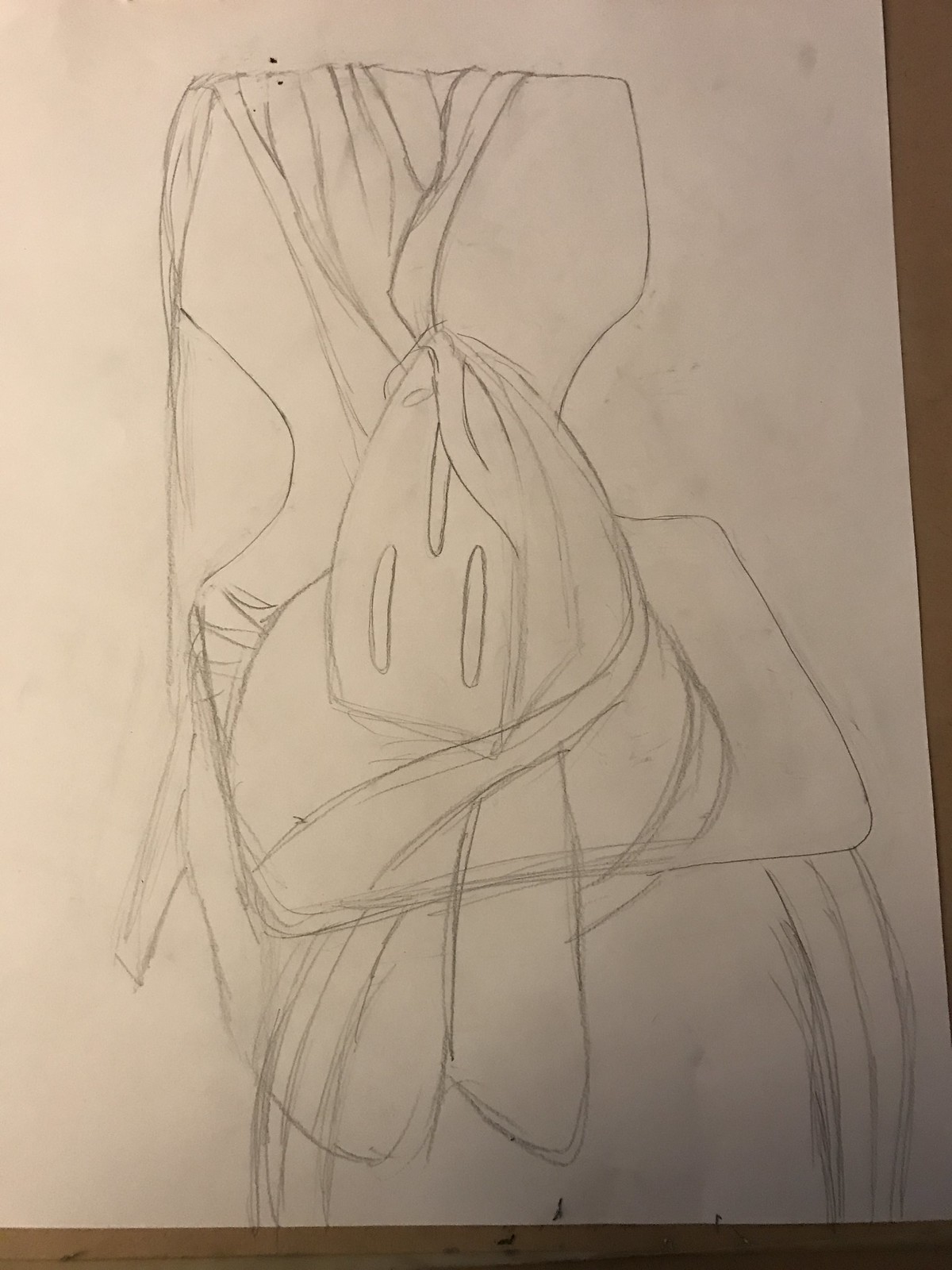This is a detailed pencil drawing on a piece of white paper, partially framed by a brown wooden tabletop visible along the upper right-hand corner and the lower edge. The paper appears slightly dirty, marked with greyish-yellowish scuffs. Central to the drawing is an image dominated by intricate pencil lines. At the bottom of the drawing, there are numerous lines—three descending on both the right and left sides.

In the middle of the image, there seems to be an upside-down face with two oval eyes, a round mouth, and a square outline around its top. Above the face, what could be interpreted as a hat or helmet is detailed, with strokes suggesting something akin to a scarf draped down. On the left side of the image, there is an element that resembles a high-heeled shoe, which could potentially indicate two shoes linked together.

Additionally, some interpretations of the drawing suggest the image might depict a chair with a cloth draped over it, possibly accompanied by an iron, showcasing the vent areas typical of a clothing iron. This artistic portrayal leaves much to the viewer's imagination with its multiple potential interpretations and rich line work.